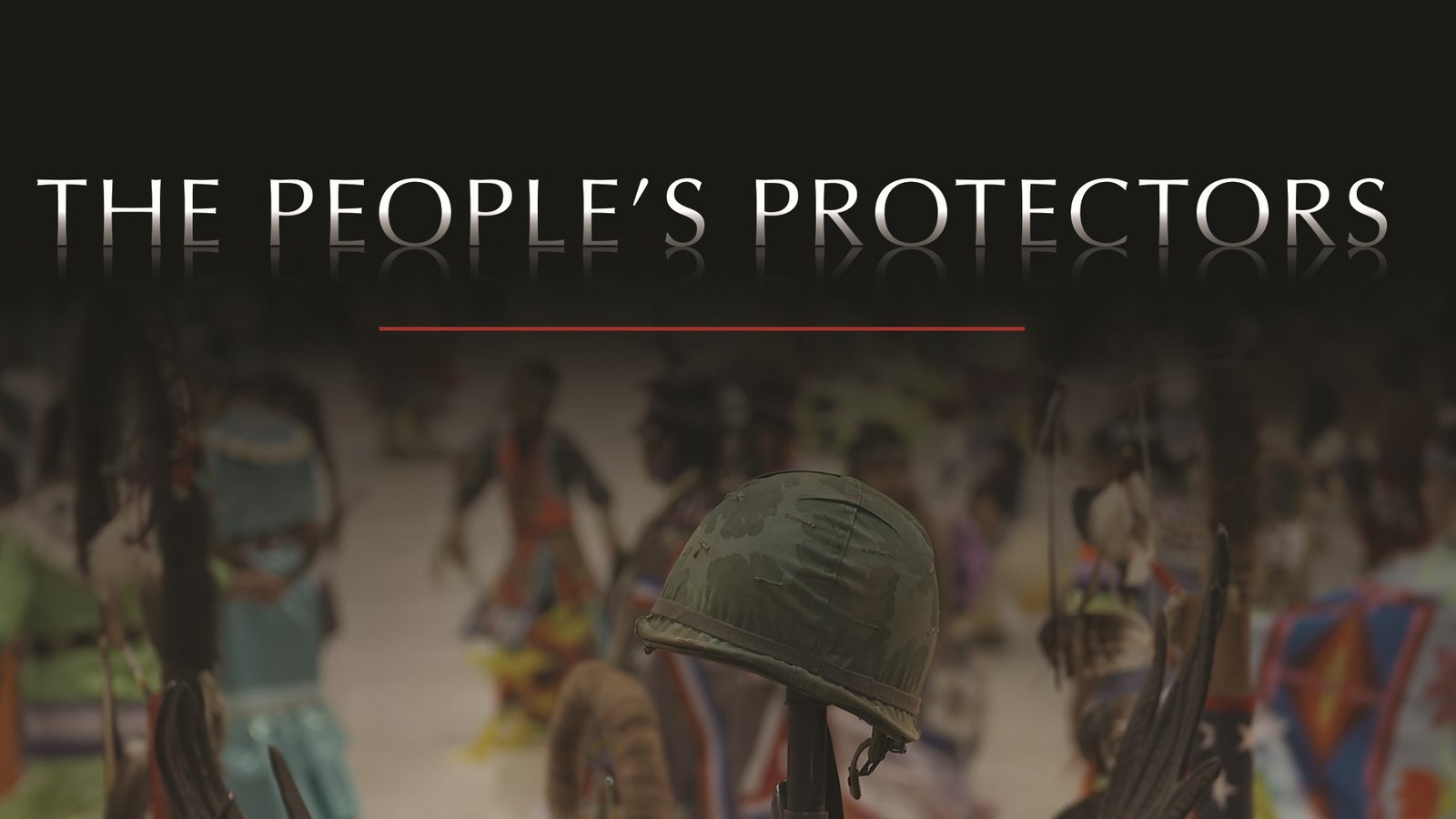In the image, the words "THE PEOPLE'S PROTECTORS" are prominently displayed at the top in white capital letters. These striking letters appear against a dark background, with a reflective effect beneath them. Directly below this phrase, a thin red line spans across the image. The central focus of the lower part of the image is a soldier's helmet, colored green, placed on top of a rifle, which is vertically positioned. This setup is akin to a battlefield cross, symbolizing fallen soldiers.

Flanking the helmet and gun are structures resembling wings, adding an element of reverence and protection. The background is quite blurry, but it depicts a group of indigenous people, possibly African or Native American, dressed in traditional, vibrant attire, with colors including green, blue, white, yellow, and red. They appear to be engaged in a dance or ceremony, contributing to a dynamic, yet indistinct backdrop. On the right side of the image, there's a white item featuring a red and blue design at its center, though its details are not entirely clear. The overall composition suggests a solemn tribute to soldiers and the communities they protect, set against a culturally rich and respectful scene.